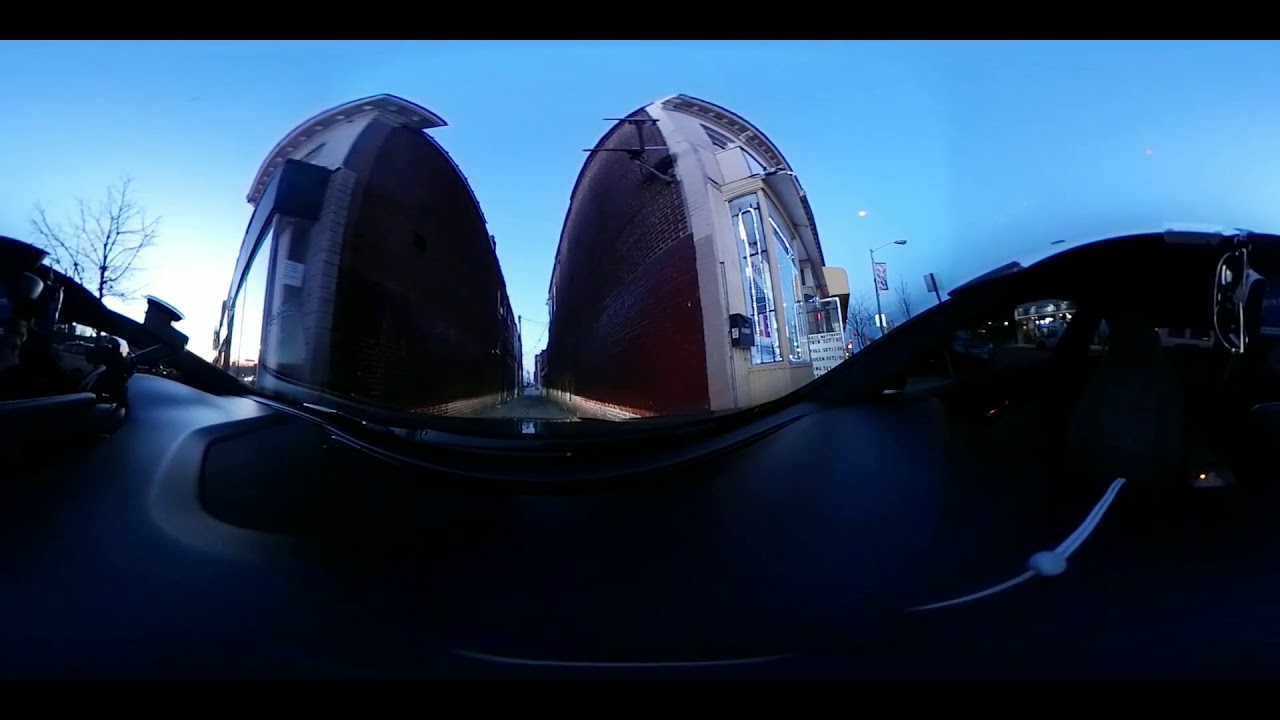The photo appears to be taken from inside a vehicle, looking out through a heavily distorted windshield, reminiscent of a 360-degree image flattened into a two-dimensional view. This distortion makes the vehicle's dashboard appear squished in the middle while stretched and warped to the sides. In front of the car, two tall, gray buildings with brick interiors align an alleyway or public road, though the curvature of their structures appears unnatural due to the photographic distortion. The view reveals street lights, some with pale moon-like dots above them, suggesting approaching twilight. To the left, a leafless tree is visible, while the right side shows multiple signs, windows, and additional buildings in the distance, partially obscured by the windshield's curve. The sky is transitioning to evening, still tinged with blue, further setting the scene.